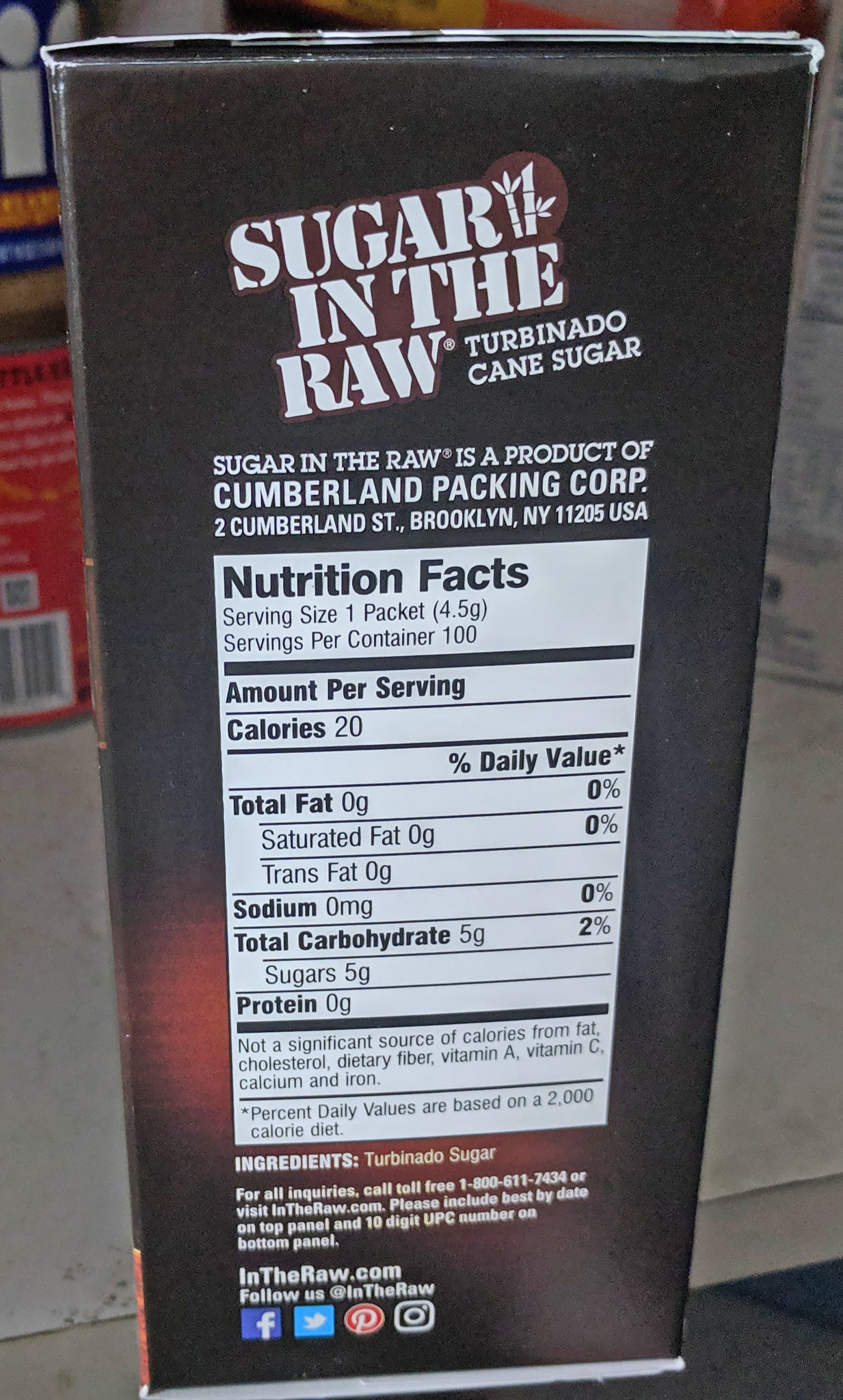Close-up of a "Sugar in the Raw" product box highlighting the nutritional information on the side. The box features a brown design with prominent bold white text stating "Sugar in the Raw" at the top, followed by smaller text that reads "Turbinado Cane Sugar." Below, there is a note indicating the product is from Cumberland Packing Corp, located at Cumberland Street, Brooklyn, New York, 11205 USA. The Nutrition Facts section, enclosed in a white box, lists details such as serving size, servings per container, and nutritional content per serving. Each serving contains 20 calories per packet, with 0 grams of total fat, saturated fat, trans fat, and sodium. The total carbohydrate content is 5 grams, all of which are sugars, and the product contains 0 grams of protein. The sole ingredient listed is Turbinado sugar.